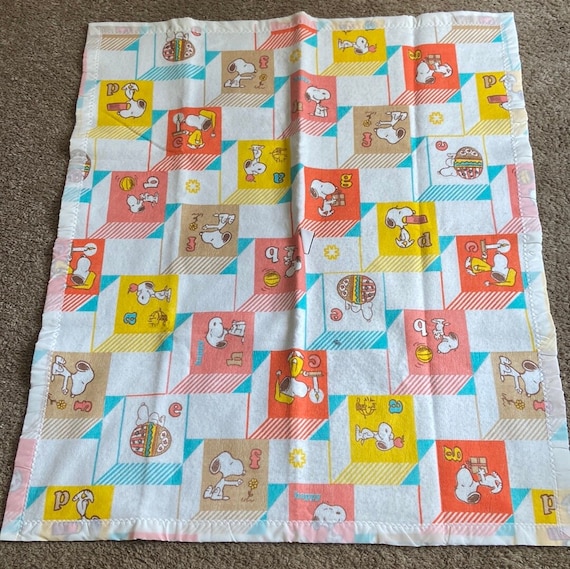This image depicts a flannel baby blanket laid out flat on a beige or taupe-colored carpet. The blanket has a white background and features a checkered pattern with different colored blocks, primarily yellow, orange, red, and beige. Each block showcases Snoopy from the Peanuts series in various poses and activities, and some blocks also feature Woodstock. Each block with Snoopy integrates a letter from the alphabet, creating an educational and playful design. Snoopy is seen performing an array of actions: carrying a present, pointing to a flower, holding a candle while wearing a nightcap and yellow pajamas, standing next to an Easter egg, and interacting with other small objects. The alternating blocks are white and serve as a contrast to the colorful blocks. The blanket's edges are bordered with a white satin strip, and the material appears thin yet very soft, ideal for a baby's comfort.